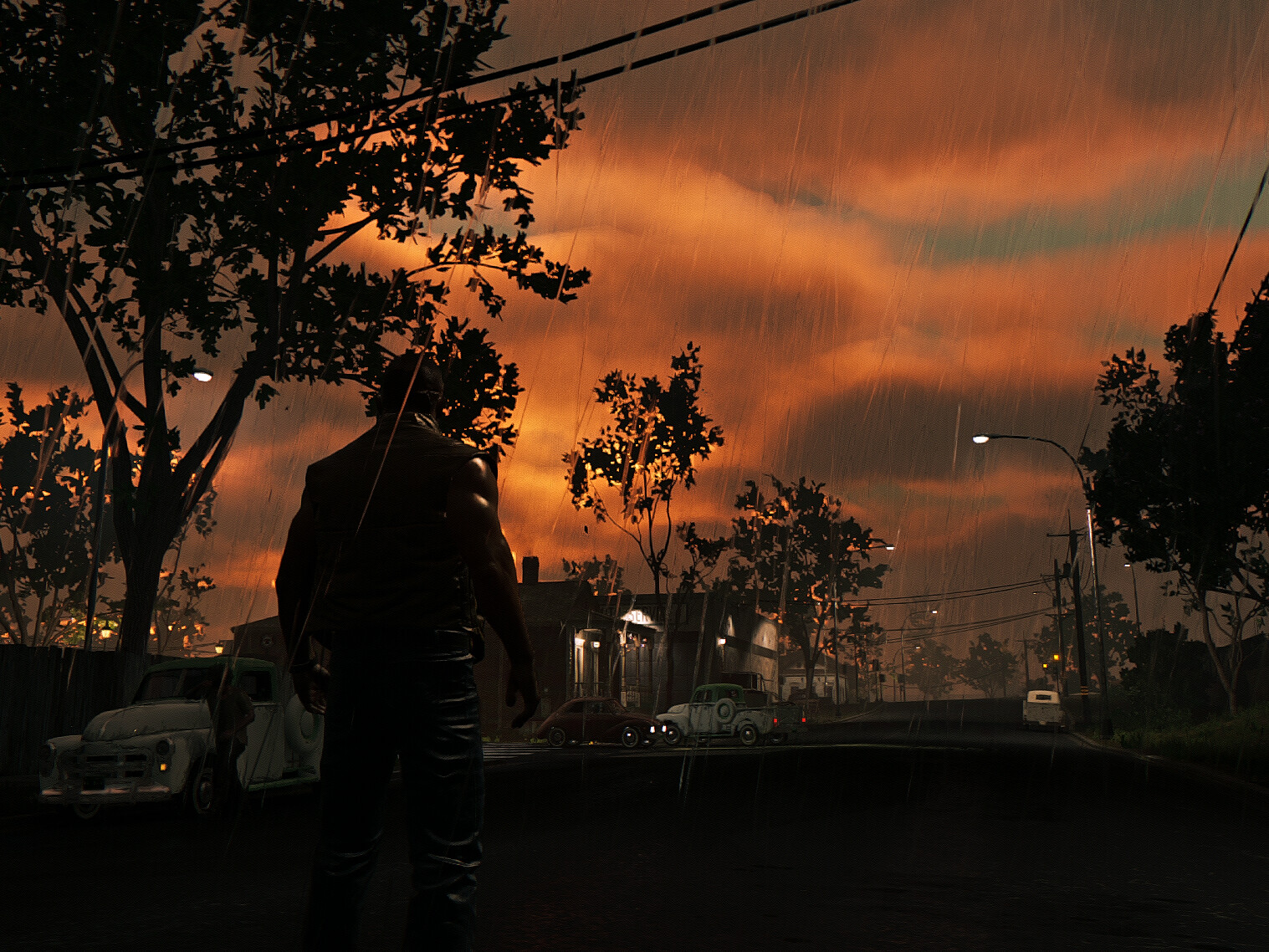This image appears to be a screen capture from a video game or a digital art painting depicting a rainy evening street scene. The viewer's perspective is eye-level, looking down a road under a dark, stormy sky with a mix of dull light blue, gray, and reddish-brown clouds suggesting the sun is setting. Raindrops are visibly falling, adding to the overall moody atmosphere. Streetlights are sparsely lit, with one prominent street light curving from the right side of the image.

On the right side, the street is bordered by small patches of grass, power lines, and a tree. Near the streetlight, there is a gray car, and further back towards the center-left of the image, more power lines and poles stretch across the scene. In the bottom left, the outline of a man is discernible, standing beside a vintage white truck with a person walking nearby. He wears a sleeveless shirt, revealing muscular arms, and black pants. The silhouette blends against the dark background with light from the streetlights providing some contrast.

Further ahead, in front of the man, a row of houses with illuminated windows line the street, flanked by several trees. Several cars, including a small car and a truck, are parked along the street. The sky above is tumultuous, with ominous, stormy clouds and occasional patches of faint blue peeking through, intensifying the scene's dramatic atmosphere.